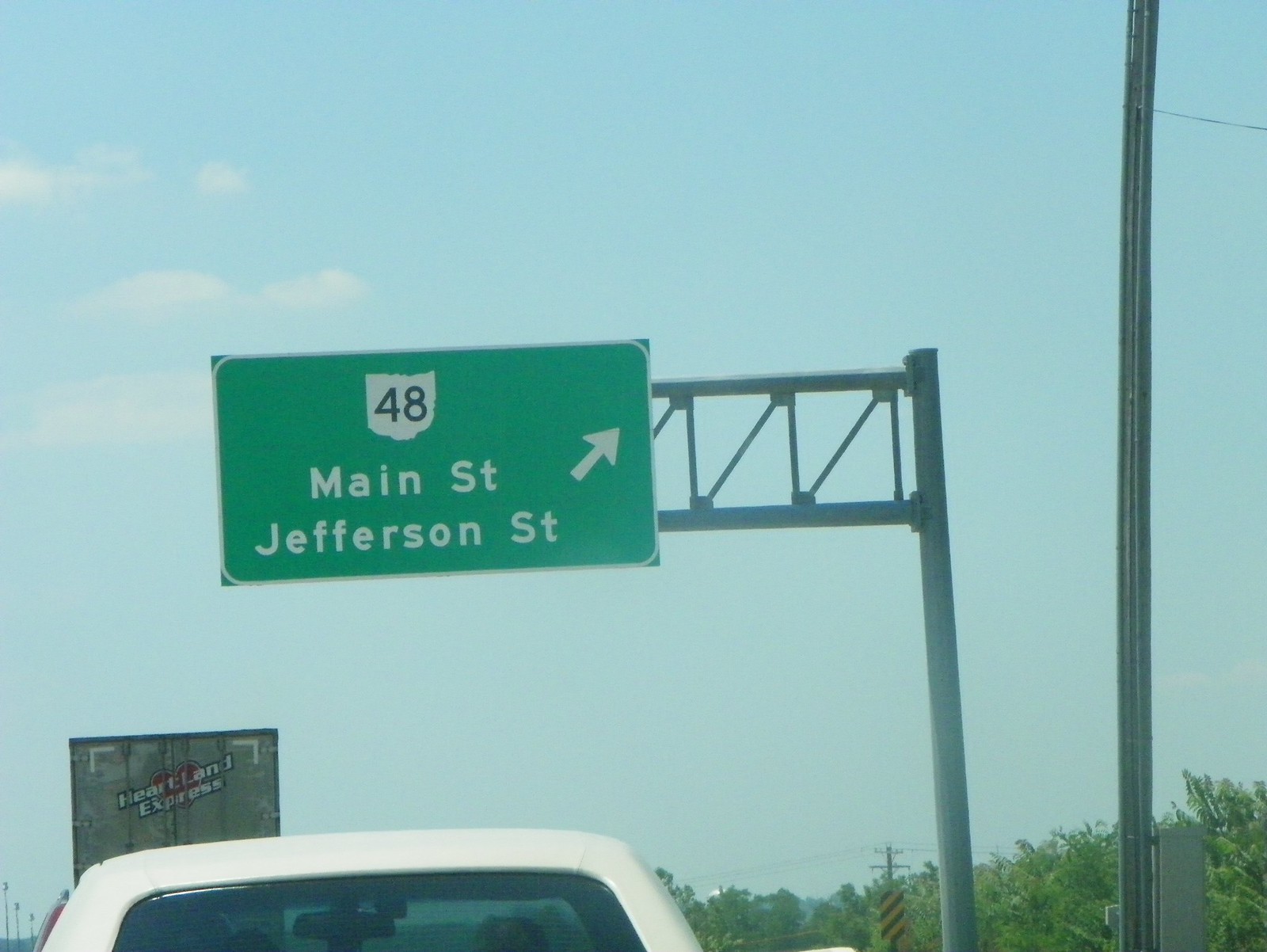This photograph captures a highway scene where the vehicle from which the photograph is taken approaches an exit onto Highway 48. The exit leads to Main Street and Jefferson Street. The scene is marked by the presence of a bridge or overpass that the exit will follow. At the lower edge of the image, there is a diagonal warning sign with red, yellow, and black stripes that typically indicates the right side of a bridge or overpass.

Dominating the right side of the frame is a utility pole, which stands near the green exit sign suspended above the interstate. This sign features a right arrow pointing toward Main Street, ultimately leading to Jefferson Street.

The background of the image is characterized by an overcast sky, setting a somewhat gloomy tone. Near the bottom of the photograph, a tree line is visible, adding a touch of nature to the otherwise urban setting. 

Traffic-wise, the vehicle is closely following an 18-wheeler, or semi-truck, as well as a white pickup truck, with the latter's tailgate and cab clearly visible in the frame. This detailed scene provides a snapshot of a typical moment on the road, just before taking a critical exit.